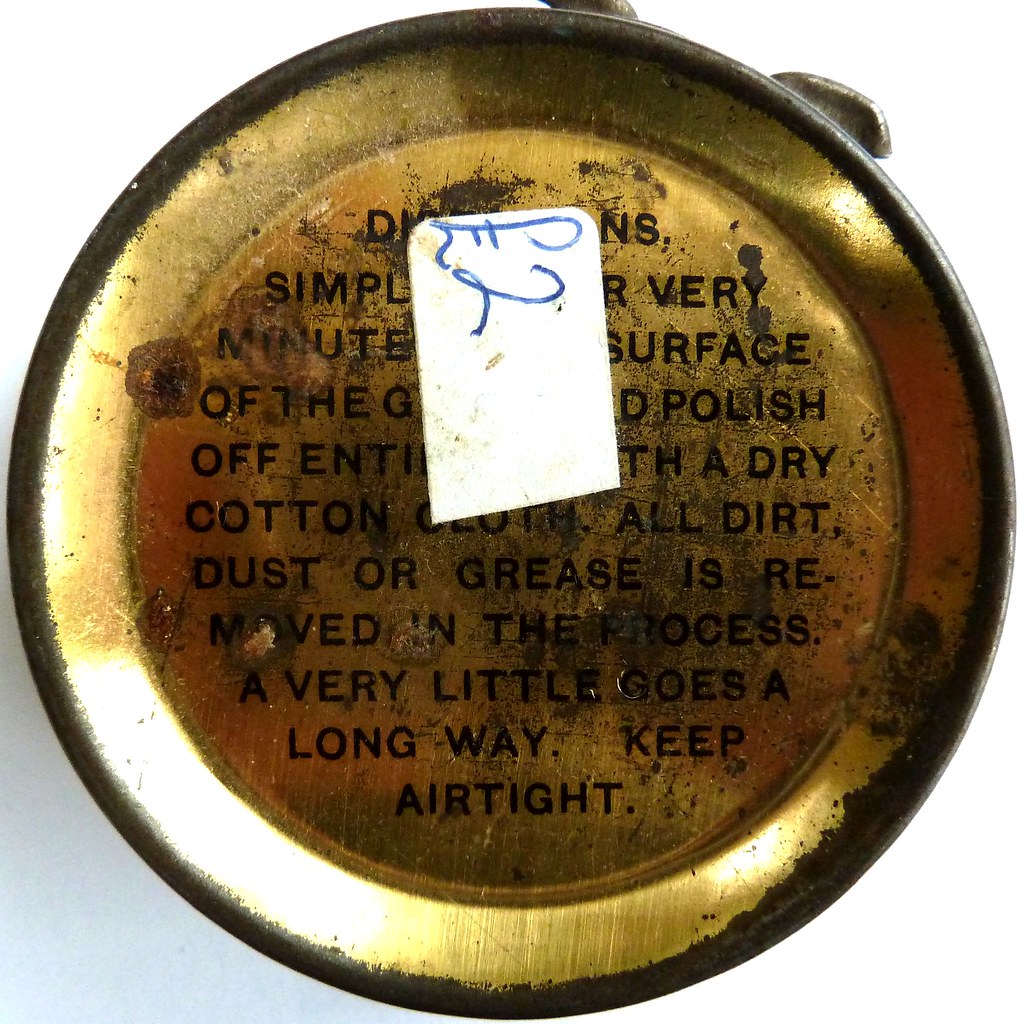This color photograph shows a detailed close-up of the bottom of what appears to be an antique or vintage metal tin, most likely a shoe polish tin, with a copper hue. The tin displays noticeable wear, including rust and patina, indicative of its age. A price sticker, reading "two pounds," partially obscures the text, which includes instructions about using the polish: "polish off entirely with a dry cotton cloth, all dirt, dust, or grease is removed in the process. A very little goes a long way. Keep air tight." The scene is composed from a top-down angle, emphasizing the tin against a white background, which might suggest a retail display setting. Additional elements like hints of gold, black, blue, and silver can be observed, potentially from the tin or its surrounding environment. The photo captures imperfections such as discoloration and small brown or black specks, reinforcing the vintage nature of the piece.